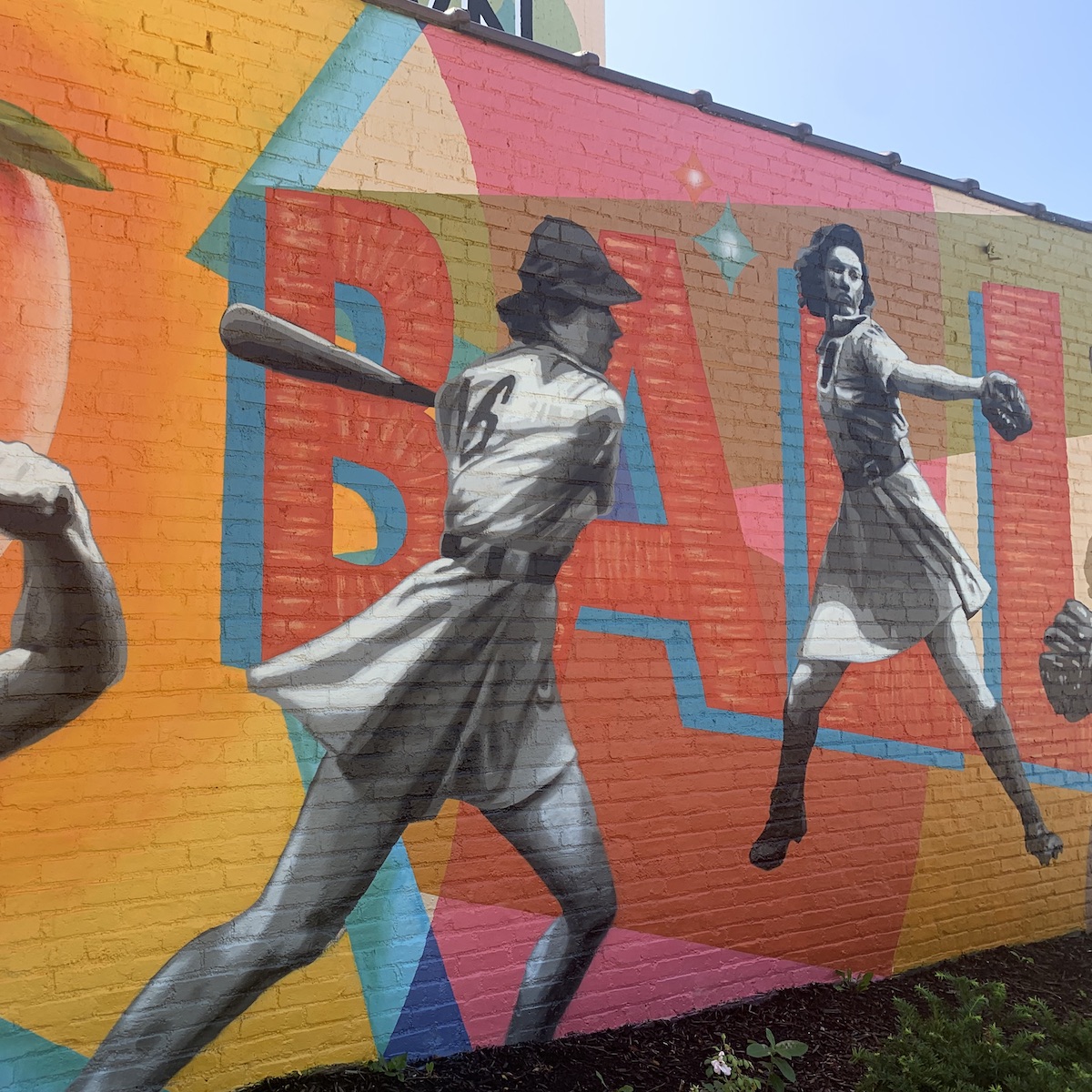The image features a vibrant and detailed mural painted on the side of a brick building. Dominantly, the backdrop of the mural showcases the word "BALL" in striking red letters. The vivid artwork, primarily in bright yellow with bursts of pink, blue, and red designs, highlights two women engaged in a baseball scene, likely paying homage to the film "A League of Their Own," celebrating female empowerment in sports. Leftmost in the mural, a woman dressed in a traditional dress-style baseball uniform with black cleats and tall black socks is captured mid-swing with a bat. Adjacent to her, another woman, poised for action, readies to pitch with a mitt on her left hand. The overall mural is energetic and nostalgic, evoking a sense of historical dedication to women's roles in baseball. In the very left corner, partially visible, is the forearm and bicep of another figure, adding to the dynamic composition of the scene.